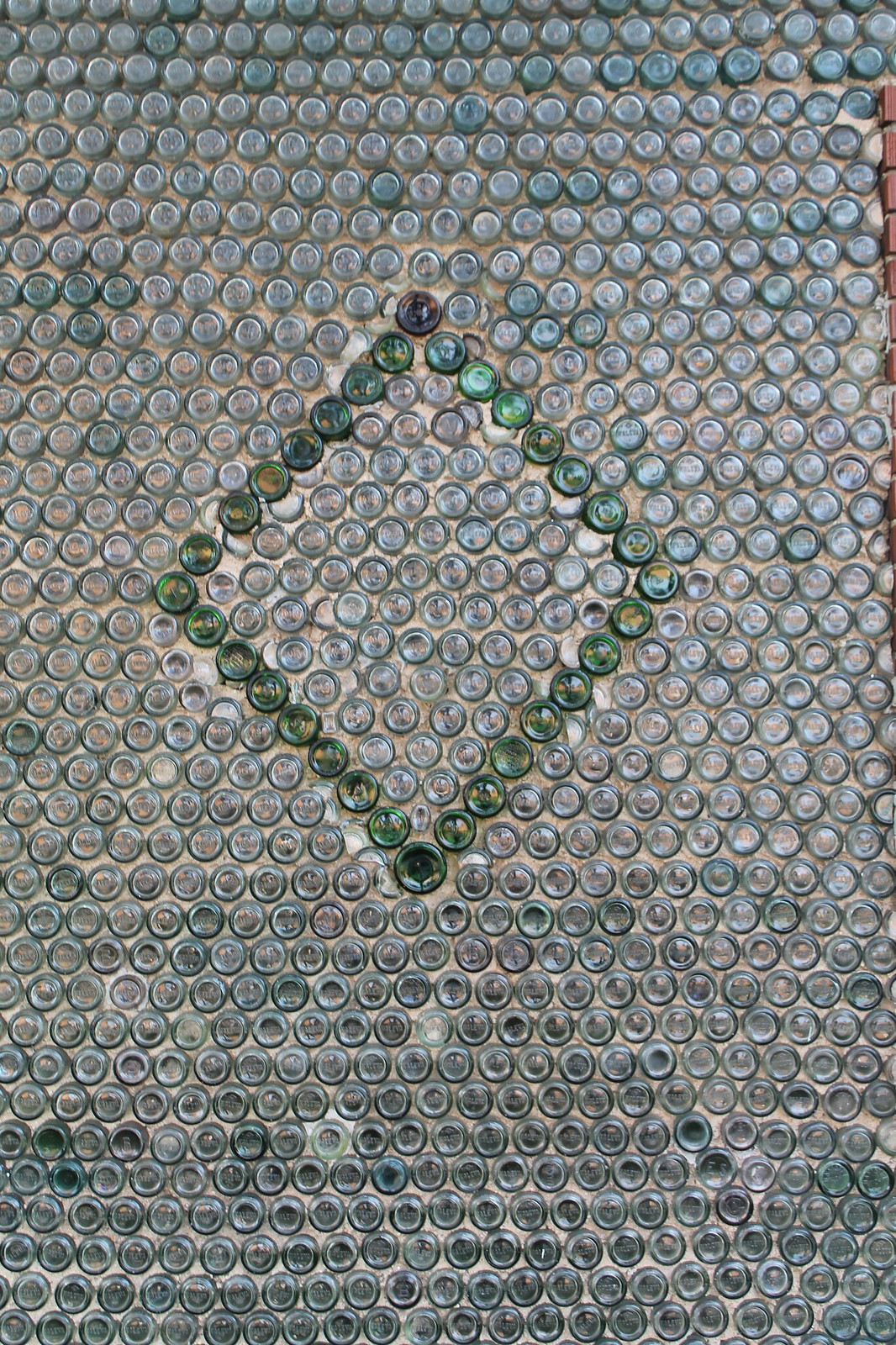The color photo depicts a mosaic made from hundreds of round objects embedded into a light-colored cement wall, located adjacent to a brick wall on the right. The mosaic elements resemble bottle caps or perhaps the bottoms of bottles, many of which are clear or have faded writing, arranged meticulously in rows. The predominantly gray background is accentuated by a striking green diamond shape in the center, formed by these green circular pieces. There's a range of colors visible, including clear, light blue, darker blue, gray, black, gold, and various shades of green. The overall appearance suggests a thoughtfully designed piece of art viewed from above, with the diamond shape providing a focal point amidst the densely packed round decorations.